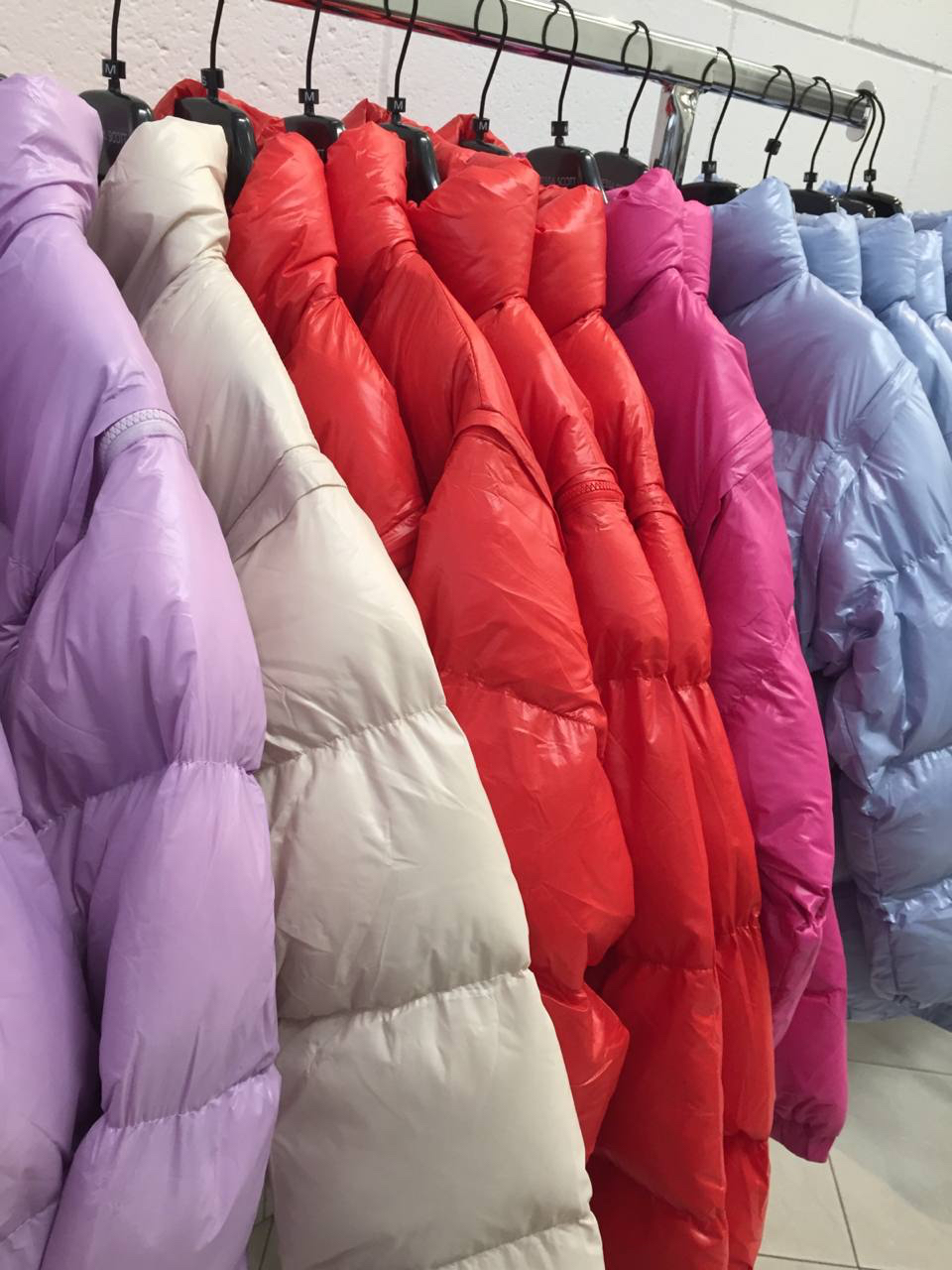This image depicts a row of puffy winter coats hanging on a long, metallic rack with hooks. Each hook is black plastic with a silver metal hook. The floor beneath the rack is white, suggesting a clean, possibly showroom environment. The sequence of the coats from right to left is as follows: three silvery grey coats, two dull pink ones, four vibrant red ones, one off-white coat, and finally a shimmering purple coat at the very front. The coats are made of a shiny, high-quality material, giving them a full and luxurious look. They all appear to be the same puffer style, designed for warmth with thick insulation. The overall arrangement and the pristine setup hint that the image might have been taken in a retail space or before a fashion show.